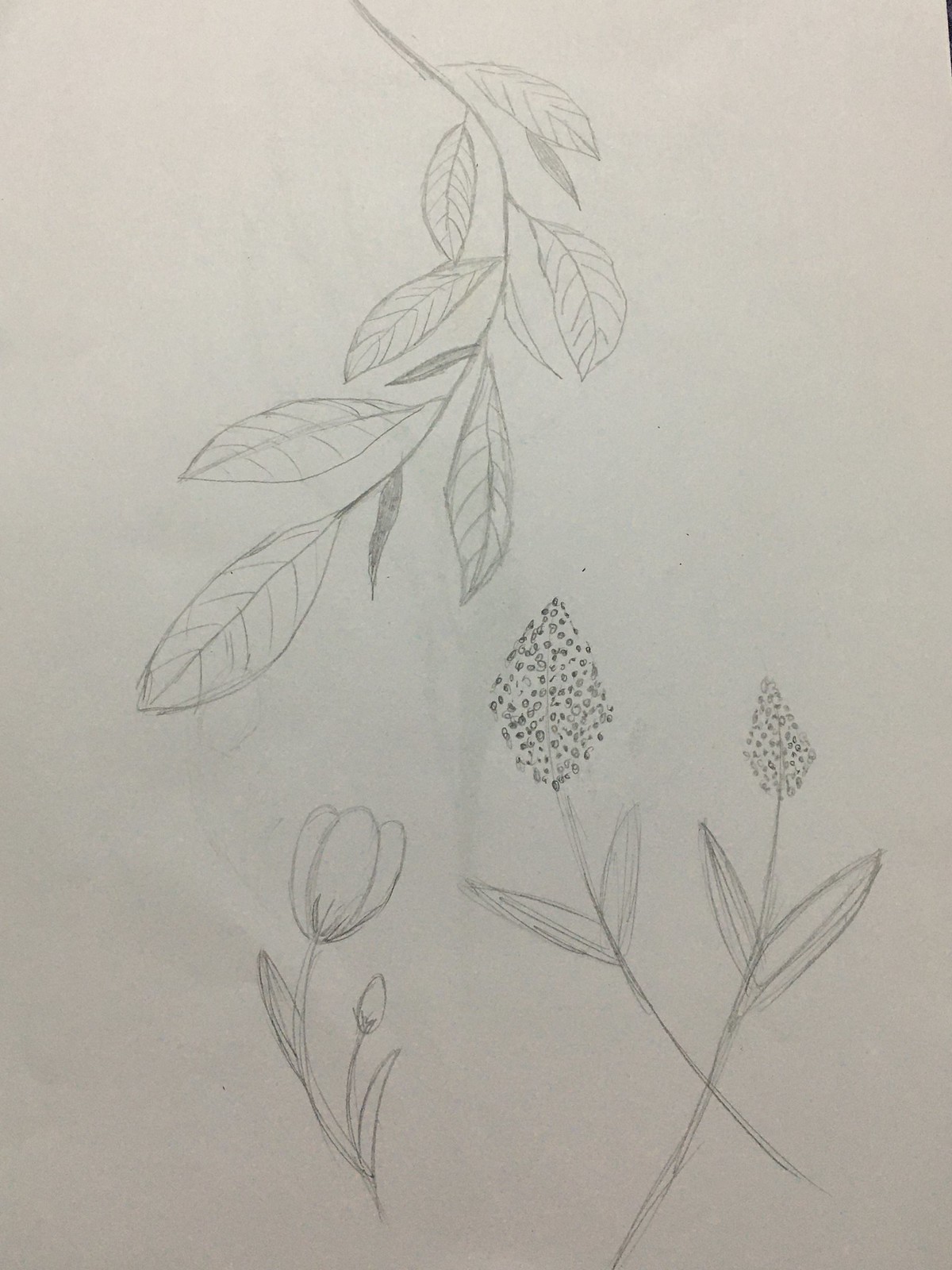This image is a delicate pencil sketch on a piece of paper with a pale lavender-gray hue. The floral scene is rendered in a very light gray pencil, giving it an ethereal quality. The composition begins at the bottom right corner, with two slender stems crossing each other. Each stem bears two pointed leaves, and the flowers on these stems are teardrop-shaped, filled with numerous tiny dots. To the left of this pair, a single-stem tulip stands gracefully. The tulip has a prominent bloom at the top, one large leaf midway down the stem, and a new bud emerging from a shorter stem near the base, accompanied by another leaf. From the top of the page, a curved stem arches downward, adorned with several pointed leaves on either side. Each leaf is intricately detailed, with a visible central vein and smaller veins extending toward the edges. The sketch captures the delicate beauty of the floral elements with its intricate lines and subtle shading.